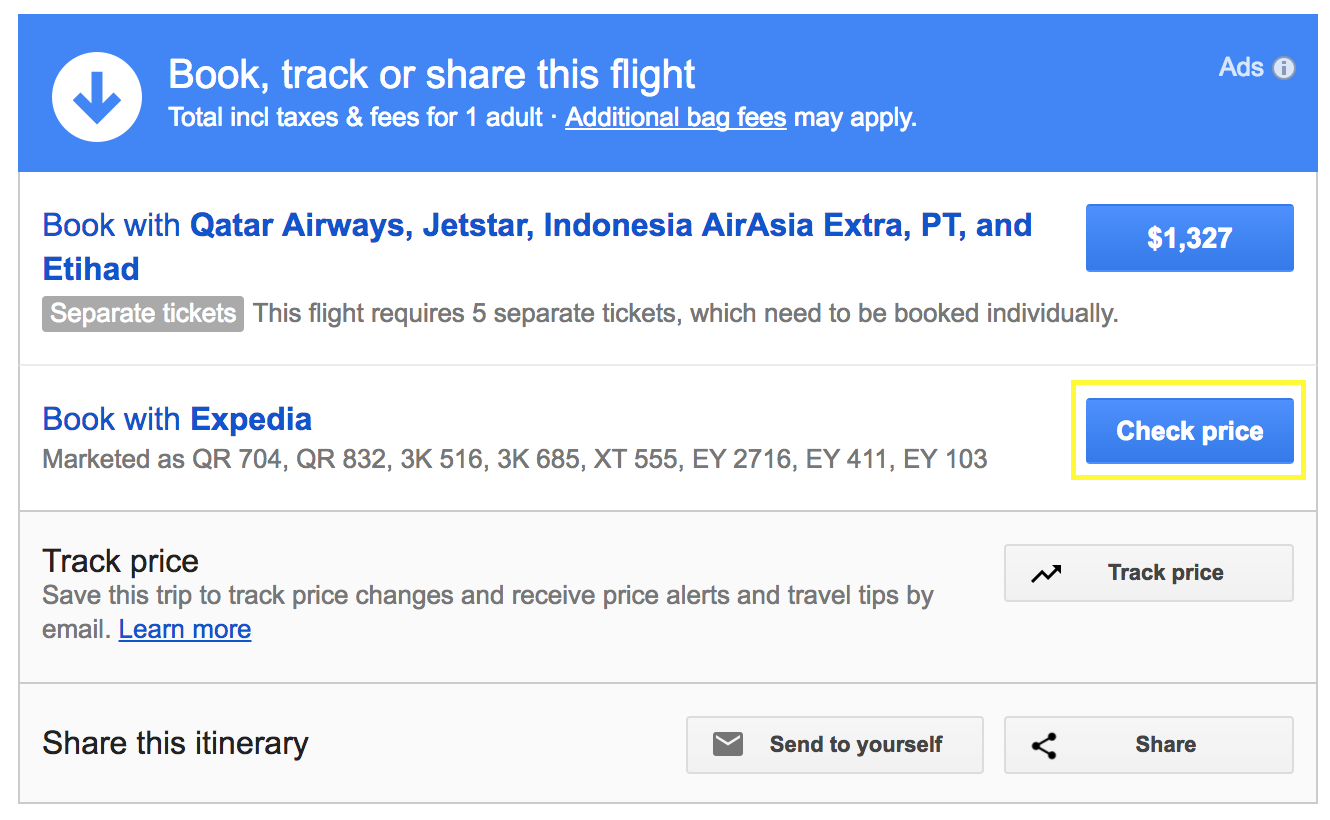This screenshot displays travel information on a website, organized for easy navigation and decision-making. 

At the top is a medium blue header featuring:
- On the left: A white circle with a medium blue downward arrow.
- Central text in white stating: "Book, track, or share this flight total, including taxes and fees for one adult. Additional bag fees may apply," with "Additional bag fees" underlined.
- On the right: The word "Ads" and a gray circle containing a dark gray eye icon.

Below the header are four line items, each set against a white or light gray background separated by thin gray lines:

1. The first line (white background) includes:
   - In blue text: "Book with Qatar Airways, Jetstar, Indonesia AirAsia Extra, PT, and Etihad."
   - A gray box with white text stating: "Separate tickets."
   - Gray text reading: "This flight requires five separate tickets which need to be booked individually."
   - On the right: A blue box with white text displaying "$1,327."

2. The second line (white background) reads:
   - In blue text: "Book with Expedia."
   - Beneath in gray text: Flight numbers "QR704, QR832, 3K516, 3K685, XT555, EY2716, EY411, EY103."
   - On the right: A blue box with white text stating "Check price," highlighted in yellow.

3. The third line (light gray background) features:
   - In black text: "Track price. Save this trip to track price changes and receive price alerts and travel tips by email."
   - "Learn more" in blue and underlined.
   - On the right: A light gray button with a black arrow pointing up and to the right, labeled "Track price."

4. The fourth line (light gray background) states in plain text: "Share your itinerary."